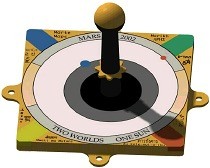The image depicts what appears to be a small board game or a game component, featuring a central, white-painted square divided into four distinct color-coded quadrants: yellow, orange, blue, and green. At the center of this square, there's a layered circular arrangement with a gray inner circle surrounded by a larger white circle, further bordered by gray and tan sections. Emanating from the center is a black pole adorned with a gold ring at its base and topped with a yellow, ball-shaped handle. The text at the bottom reads "Two Worlds One Sun." The entire board shows notable details such as blue and red dots orbiting the central circle, and attachment points that suggest the possibility of hanging or mounting the board. The quadrants and intricate central design underline its function, possibly as part of a gameplay mechanism.